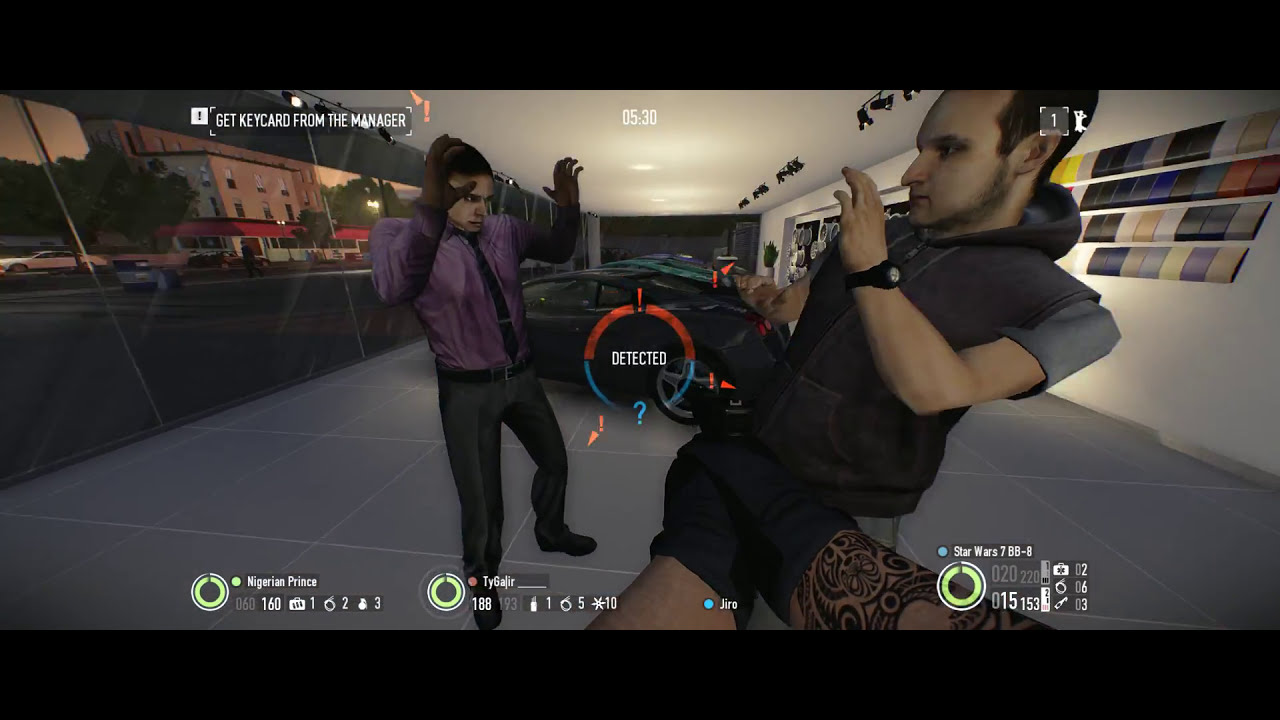This is a detailed screenshot from a first-person shooter video game, featuring a chaotic scene inside a luxurious car dealership. The player's perspective shows two gloved hands, with a tattooed right arm aiming a handgun at two NPCs. The screen includes a directive in the upper left corner stating "get key card from the manager." In the top center, "0530" is displayed, and prominently in the middle of the screen, a circle icon marked with "detected" shows an exclamation mark on top and a question mark on the bottom.

The NPC on the right, who appears to be startled, is leaning back and has lighter skin. He is dressed in a gray short-sleeved shirt with a dark gray sleeveless hoodie, suggesting he might be a guest or a customer. The main target, indicated by the directive, is a man in a purple dress shirt with a black tie and gray slacks, identified as the manager. Both NPCs have their hands raised, indicating they are either being held up or threatened. In the background, a showroom filled with supercars like Ferraris and Lamborghinis adds to the opulent setting of this intense in-game moment.